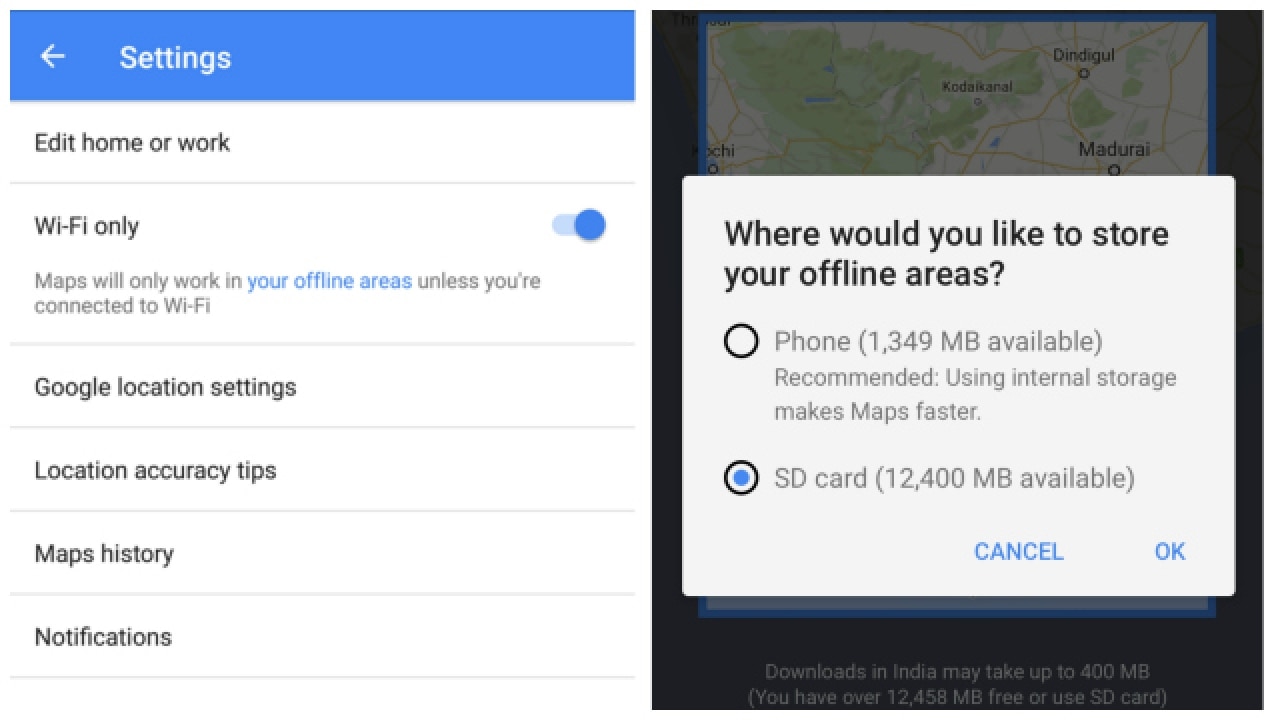In the image, a settings menu is displayed over a semi-transparent map. At the top of the screen, a blue band contains a back arrow and the title "Settings" in white text. Below this, the section "Edit home or work" is underlined, indicating it's an interactive option. A toggle switch next to "Wi-Fi only" shows that maps will only function in offline areas unless connected to Wi-Fi, and this option is currently enabled.

The central focus of the image is a pop-up titled, "Where would you like to store your offline areas?" The user can choose between "Phone (1349 MB available)" with a note that using internal storage makes maps faster, and "SD card (12400 MB available)," which is currently selected. At the bottom of the pop-up, there are two buttons: "Cancel" and "OK."

On the left side of the screen, there are additional options for "Google location settings," "Location accuracy tips," "Map history," and "Notifications." The color scheme includes predominantly blue, white, black, and gray, with subtle hints of green, yellow, and tan visible on the underlying map, though the map itself is mostly obscured by the settings overlay.